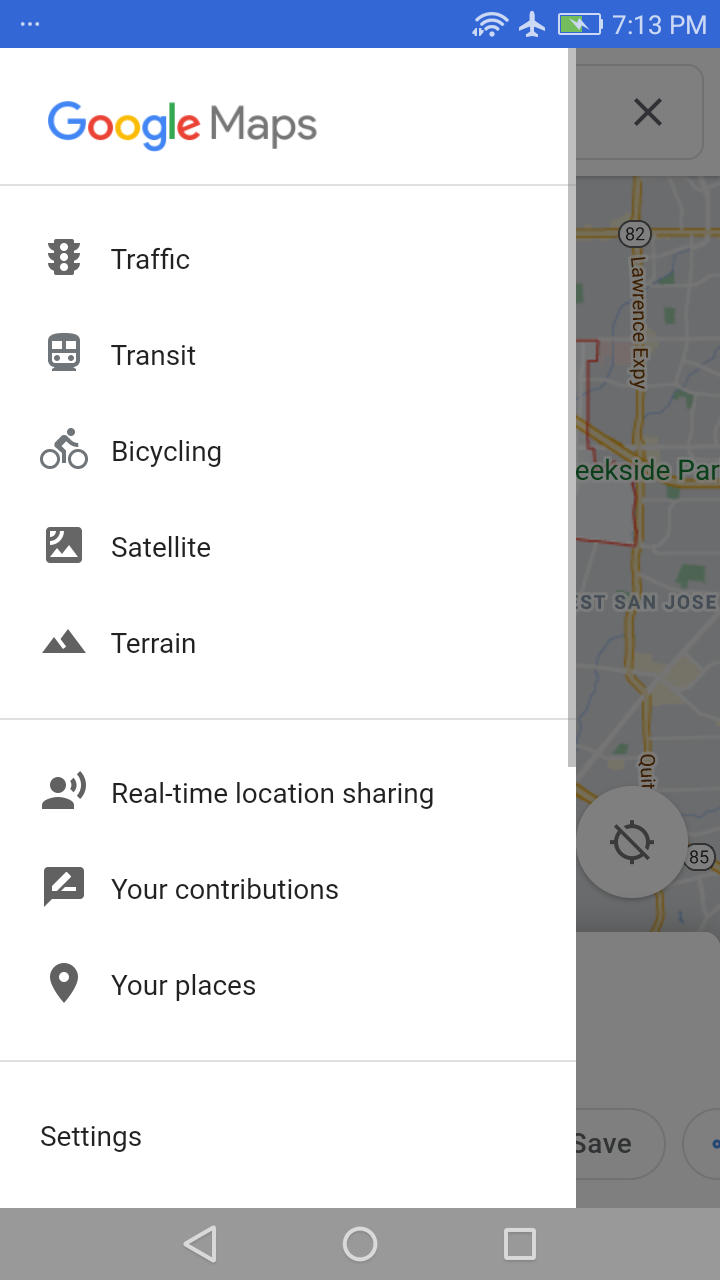A detailed screenshot from a mobile phone displaying Google Maps is shown. At the top of the screen, the Google Maps logo is prominently visible. A drop-down menu is open, obscuring a significant portion of the map, making it difficult to identify the exact city location. The menu presents several options: "Traffic" with a grey icon of a traffic light, "Transit" illustrated with a bus or sky train icon, "Bicycling" depicted by a person on a bicycle, "Satellite" marked by a grey image of the sun and mountains, and "Terrain" indicated by mountain symbols.

Below these options, the menu is divided by a grey horizontal line, leading to additional choices including "Real-time location sharing," "Your contributions," and "Your places." Another horizontal line separates these from the "Settings" option at the bottom of the menu.

Visible through the semi-transparent menu on the map are specific locations: Creekside Park, a reference to West San Jose, and Lawrence Expressway, suggesting the location is in California.

The status bar at the top of the phone screen indicates the device is in airplane mode, showing approximately 50% battery power and the time as 7:13 PM. Despite being in airplane mode, data appears to be in use.